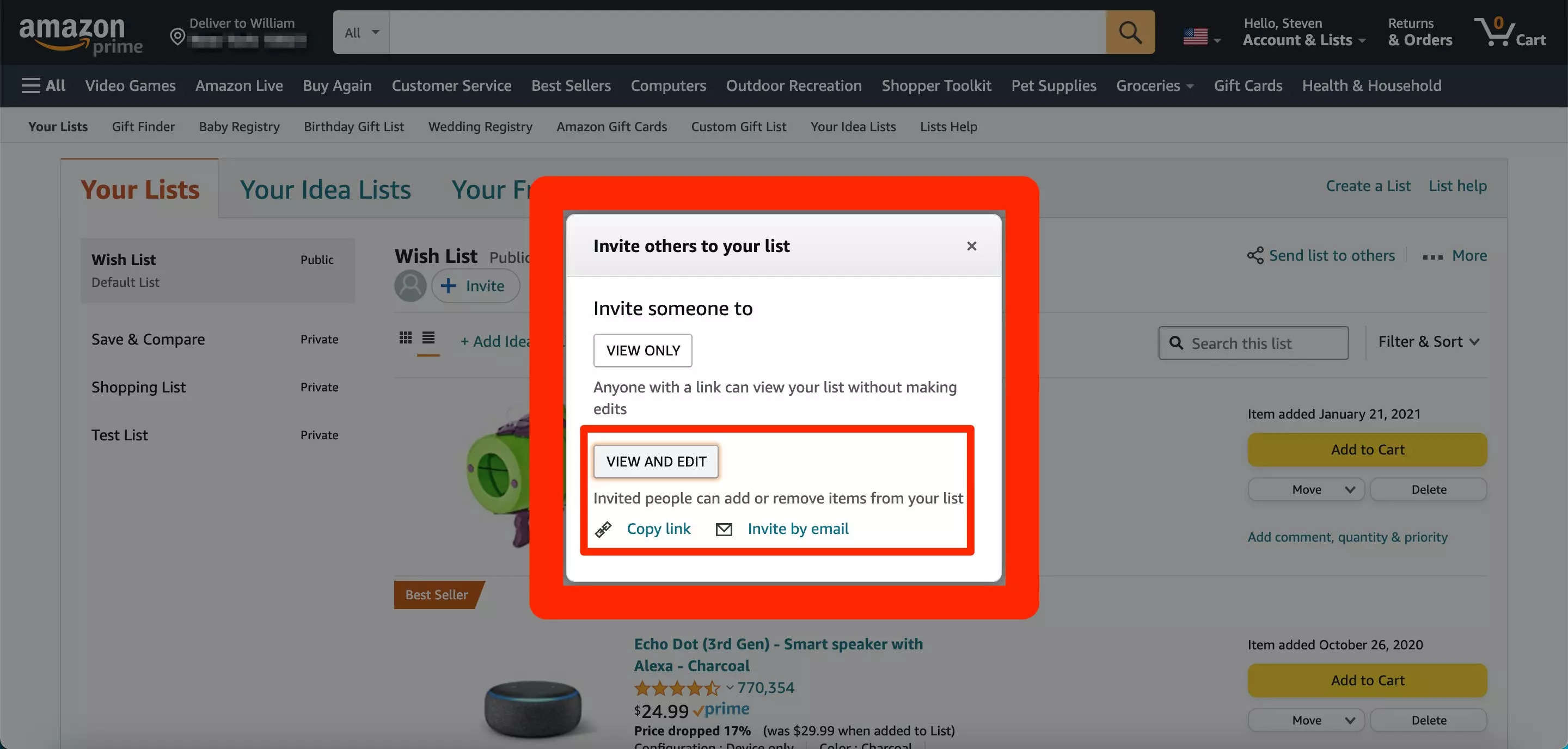This image showcases an Amazon web page characterized by its standard layout, adorned with a white background and the iconic Amazon logo prominently displayed at the top, denoting a recognizable and safe browsing spot. The upper left corner features the Amazon Prime logo, next to which lies the ubiquitous search bar, flanked by country filters, evident from the American flag, and traditional menu options including Account & Lists, Orders, and the Shopping Cart.

Beneath this standard navigation panel is a categorized menu offering quick links to departments such as Video Games, Buy Again, Customer Service, Best Sellers, Computers, For Sellers, Gift Cards, Health & Household. This is followed by another tier of links, facilitating access to Gift Finder, Wedding Registry, various gift lists, and more.

To the left, a user's personalized section is visible, comprising 'Your List' that features the wish list and shopping cart, alongside 'Your Idea List.' The image partially cuts off another tab due to a prominent red-bordered box centrally positioned on the page, intended to capture immediate attention.

This central box slightly greys out the rest of the content, thereby accentuating itself. Inside, a dropdown menu titled "Invite others to your list" sits on top, allowing users to invite others either for view-only access or with view and edit permissions. The overlay of this red-bordered box disrupts the full view of several products underneath; noticeably, a lime green device and an Amazon Echo device.

To the right of this red-bordered box, the regular Amazon page continues with options to add items to the cart along with timestamps indicating when such actions were taken. The encompassed red box with a dropdown is indicative of a collaborative feature intended for sharing and editing gift lists with others.